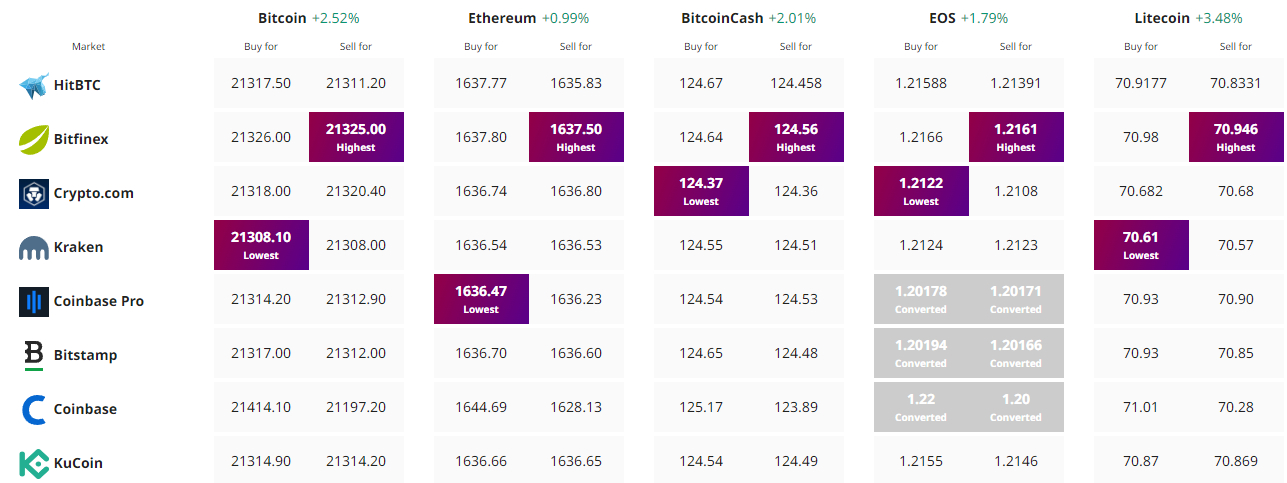This image represents a detailed cryptocurrency trading board showcasing the current buying and selling prices across various platforms. On the left-hand side, there's a list of major cryptocurrency exchanges including HIT BTC, Bitfinex (with a leaf icon), Crypto.com, Kraken, Coinbase, and KuCoin. Each platform is denoted with its respective logo.

The board is divided into five main columns, each for a specific cryptocurrency: Bitcoin (BTC) at 2.52%, Ethereum (ETH) at 0.99%, Bitcoin Cash (BCH) at 2%, EOS at 1%, and Litecoin (LTC) at 3%. Each column lists the buying ("Buy") and selling ("Sell") prices offered by each exchange platform.

Specific areas on the board are highlighted in different colors; some areas are highlighted in purple, while several sections under EOS are highlighted in a lightish gray, totaling about six sections. The numbers in each row correspond to the buy and sell prices offered by the listed exchanges for each cryptocurrency.

This comprehensive table allows users to compare the best buying and selling rates for Bitcoin, Ethereum, Bitcoin Cash, EOS, and Litecoin across these popular cryptocurrency trading platforms.